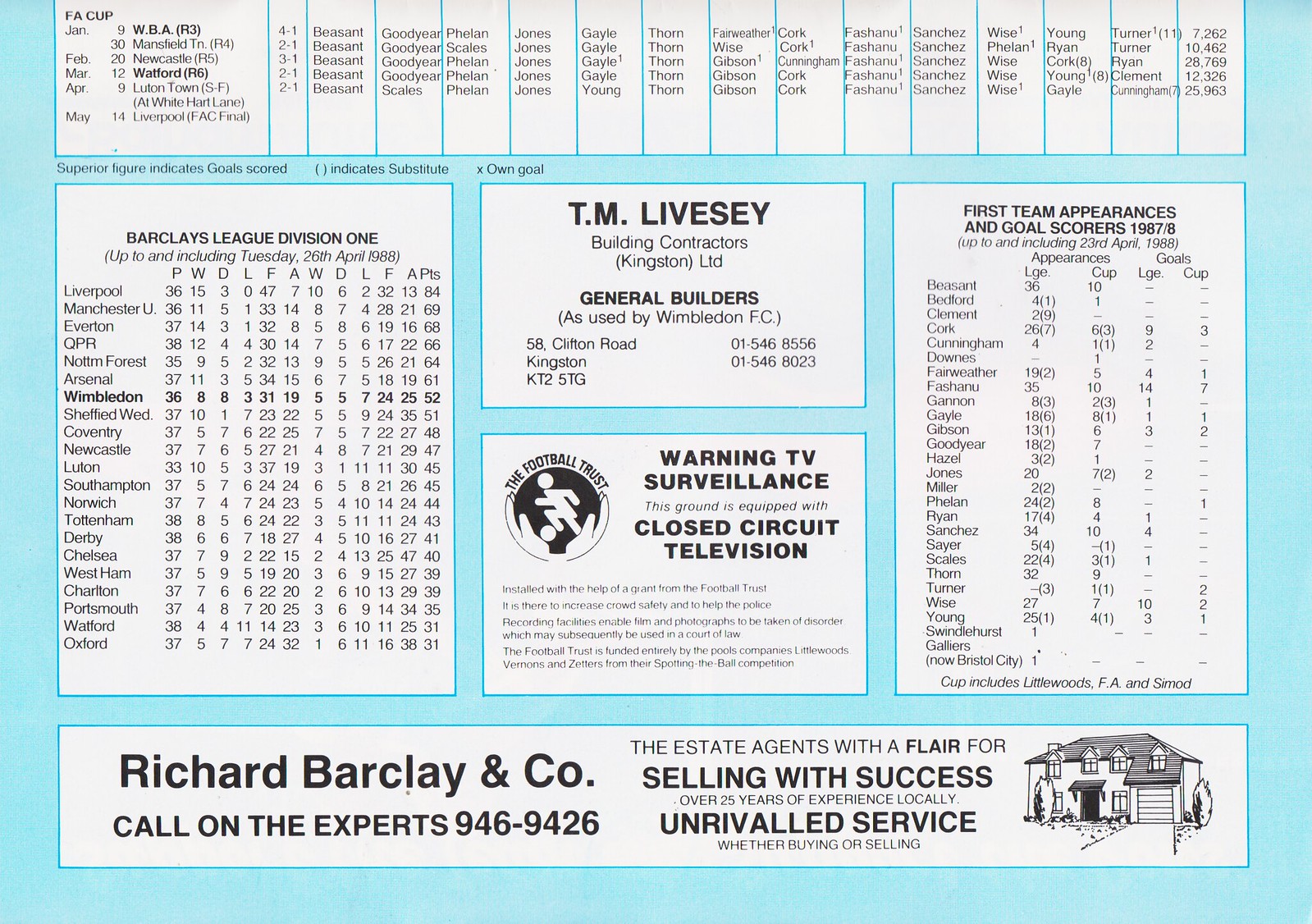In the image, there is a detailed score table, seemingly for a soccer game, prominently labeled with "FA Cup" at the top. The table is organized by months, with January, February, March, April, and May listed, highlighting important fixtures and dates. Numerous team names such as WBA, Newcastle, Watford, and Liverpool are noted. 

Under the FA Cup, the table includes player stats, relevant to Barclays League Division One, with player names such as Besant, Can, Condier, Belm, Jones, and Gale mentioned. 

In the middle, there is a prominent blue box with the text "Team Lipsy, Building Contractors (Kingston) LTD, General Builders as used by Wimbledon FC," including their address at 58 Clifton Road, Kingston, KT2 5TG, and contact numbers 01-546-8556 and 01-546-8023. The logo features a cartoon soccer player within a black circular design.

On the right side, the image has advertising content: "Richard Barclay and Company," promoted as “selling with success," and an estate agency emphasizing local expertise with "over 25 years experience" and "unrivaled service." 

Prominent warnings about TV surveillance and closed-circuit television are included for security emphasis. At the bottom of the image, "Richard Barclays and Co., called the Experts, 946-9426," is noted, next to a black-and-white depiction of a house with a black roof.

Overall, the image serves as a blend of a comprehensive scorecard and multifaceted advertisement, capturing various aspects of the soccer game details and local business promotions.